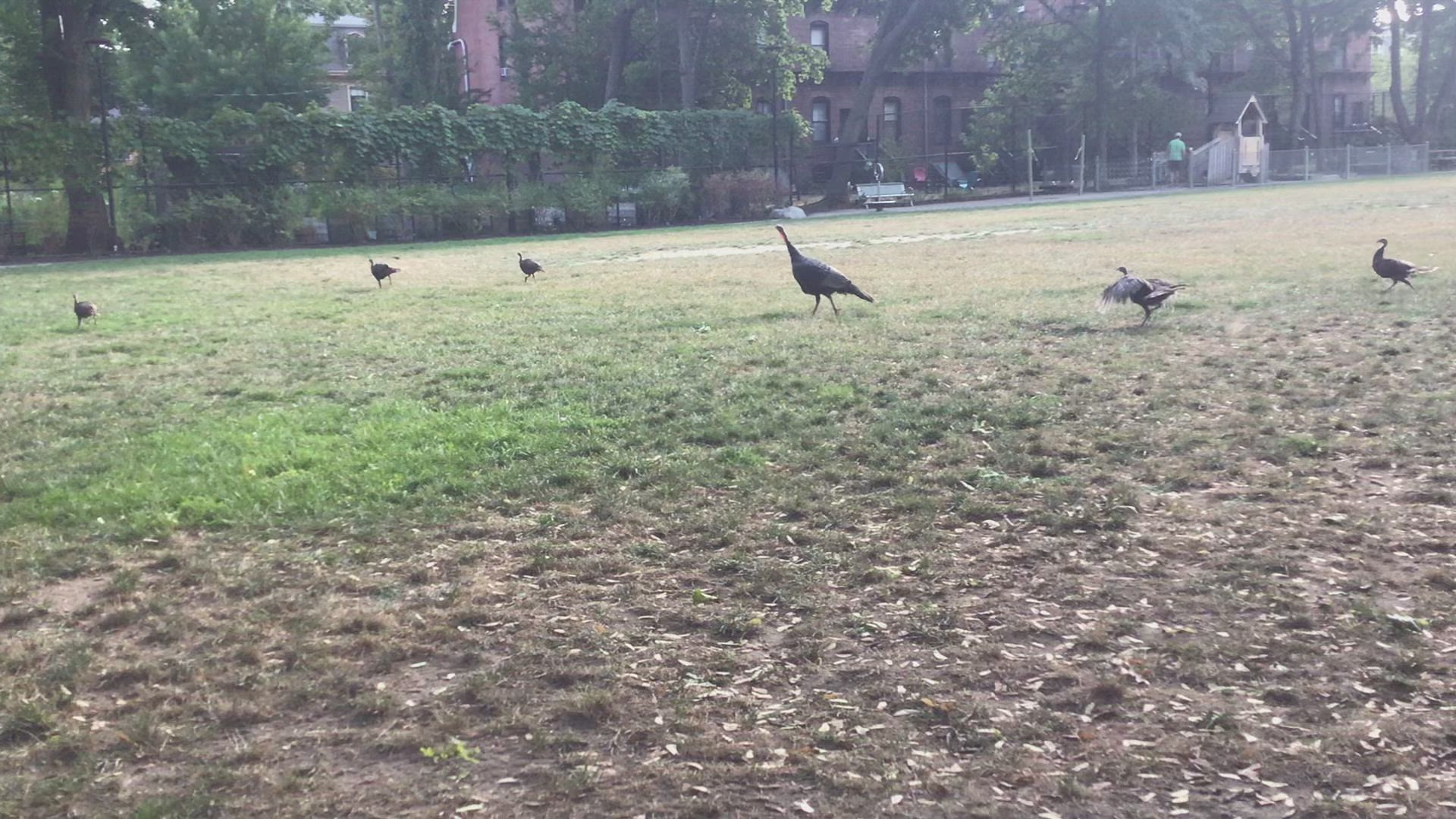This is a detailed color photograph of a large field, taken on an overcast day, giving the image a darker tone. The rectangular, horizontal image captures a scene dominated by a mostly dried, brown grassy field with sporadic green patches and a small dirt pathway off in the distance. The foreground is sparse, featuring dirt and seed pods.

Central to the image is a large wild turkey, positioned towards the center of the field, walking from right to left, with its tail pointed down. Accompanying it are five smaller birds, likely its offspring. Three of these smaller birds are in front of the turkey, while two are behind, with one flapping its wings as if rushing to catch up. 

In the background, the field extends towards a hedgerow and a brick wall. Beyond these, a large brick building, potentially several interconnected structures, stands prominently. Additionally, there is a smaller white structure with a pitched roof that might serve as an entrance or shelter. Metal fencing with ivy growing over it partially encloses the area, and another fenced section is visible where a man in a white shirt stands. Trees frame the background, adding to the depth of the scene.